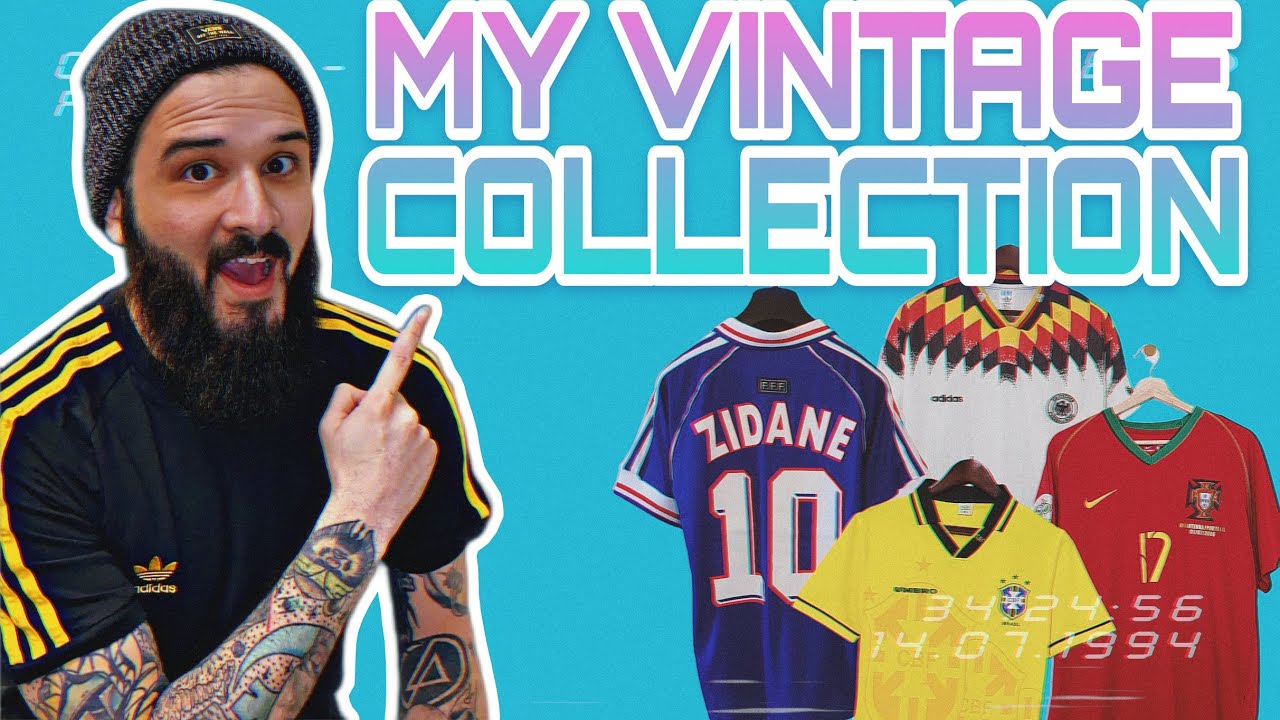This image appears to be an advertisement or YouTube thumbnail with a vibrant, baby blue background. On the left side of the image is a young man in his 20s, wearing a simple grey beanie and a black Adidas shirt with yellow stripes down the shoulders and sleeves. He has a medium-length beard, a Fu Manchu style mustache, dark eyebrows, and heavily tattooed arms featuring blue, black, red, and yellow ink. The man is pointing up towards the text "My Vintage Collection," which is displayed in a retro, rounded typeface featuring a gradient from hot pink to turquoise, outlined in white.

To the right of the man, four prominently displayed jerseys are visible. The first is a blue sports jersey displaying the name "Zidane" and the number 10. Behind it is a white Adidas jersey adorned with black, red, and yellow diamond shapes. The third jersey is yellow and plain, likely representing a Brazilian soccer theme. The fourth jersey, in red, features the number 17, a Nike logo, a green collar, and an emblem, giving it a Spanish soccer vibe. Additionally, superimposed across the red jersey is a sequence of numbers: 3424-5614071994, resembling a time stamp. The entire setup exudes a lively, vintage sports collection theme.